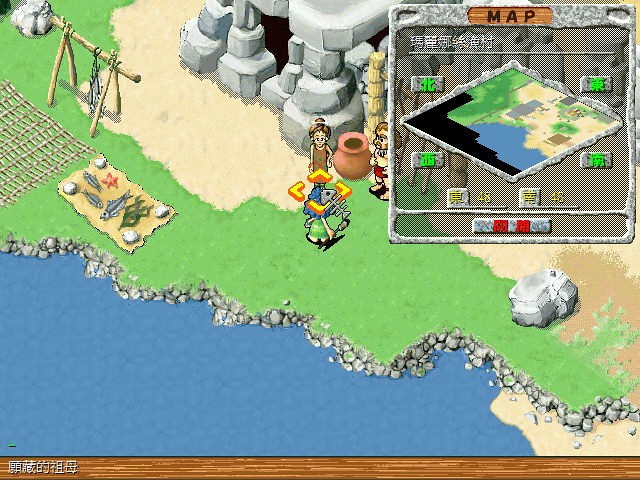In this image captured from a gameplay scene, the bottom portion showcases a rustic, wooden floor adorned with white, foreign characters. Adjacent to this floor is a body of blue water, leading to a rocky shoreline with stones in shades of white and gray, interspersed with patches of light green grass. On one side, a fishing net is visible, along with several fish laid out on a tan surface. These fish exhibit a silver-white hue, and nestled among them is a pink starfish. There’s also some green seaweed present. Additional fish are seen hanging from a wooden structure.

In the background, a stone-gray structure stands amid a sandy area. Two characters are present: a brown-haired woman dressed in brown attire, and a shirtless man in red swim trunks, sporting a mustache and brown hair. Another character with blue hair is seen carrying a club, with a fishbone icon hovering over their head; this character is dressed in green and has a yellow box over their head.

At the top of the image, there is a stone-colored map displaying an aerial view with green highlights.